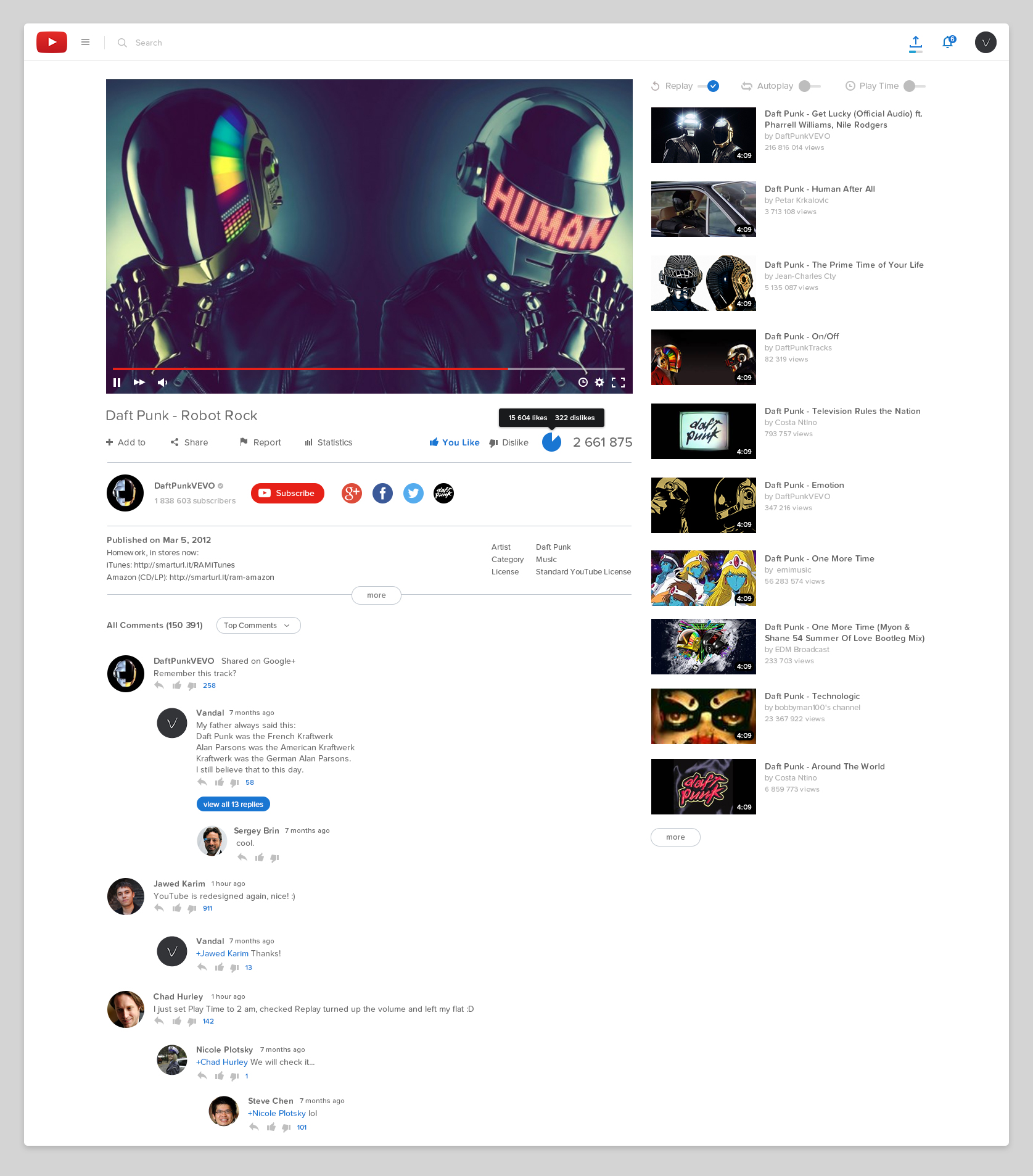The image showcases the YouTube application open on a device, playing a music video titled "Robot Rock" by Daft Punk. In the video thumbnail, two figures dressed in black leather jackets, black gloves, and bike helmets are featured. The person on the left is wearing a helmet adorned with music equalizer bars in red, green, and yellow. The individual on the right sports a glossy black helmet with a blue visor displaying the word "Human" in red letters. The video is uploaded by the channel "Daft Punk VEVO."

The top comment reminisces, "Remember this track from Daft Punk VEVO," to which a user named Vandal replies, "My father always said Daft Punk was the French Kraftwerk. Alan Peterson was the American Kraftwerk. Kraftwerk was the German Alan Peterson. I still believe that to this day." Other comments include Jode Kidding exclaiming, "YouTube is redesigned again," Vandal responding, "Thanks," Charge Hardly sharing, "I set playtimes to 2 a.m., checked replay, turned up the volume, and left my flat," Nicole stating, "We'll check in," and Steve Chen simply saying, "LOL."

On the right side of the screen, there are additional playlists from Daft Punk, featuring tracks like "Get Lucky," "Human After All," "The Prime Time of Your Life," "Television Rules the Nation," "Emotion," "One More Time," "One More Time Again," "Technologic," and "Around the World."